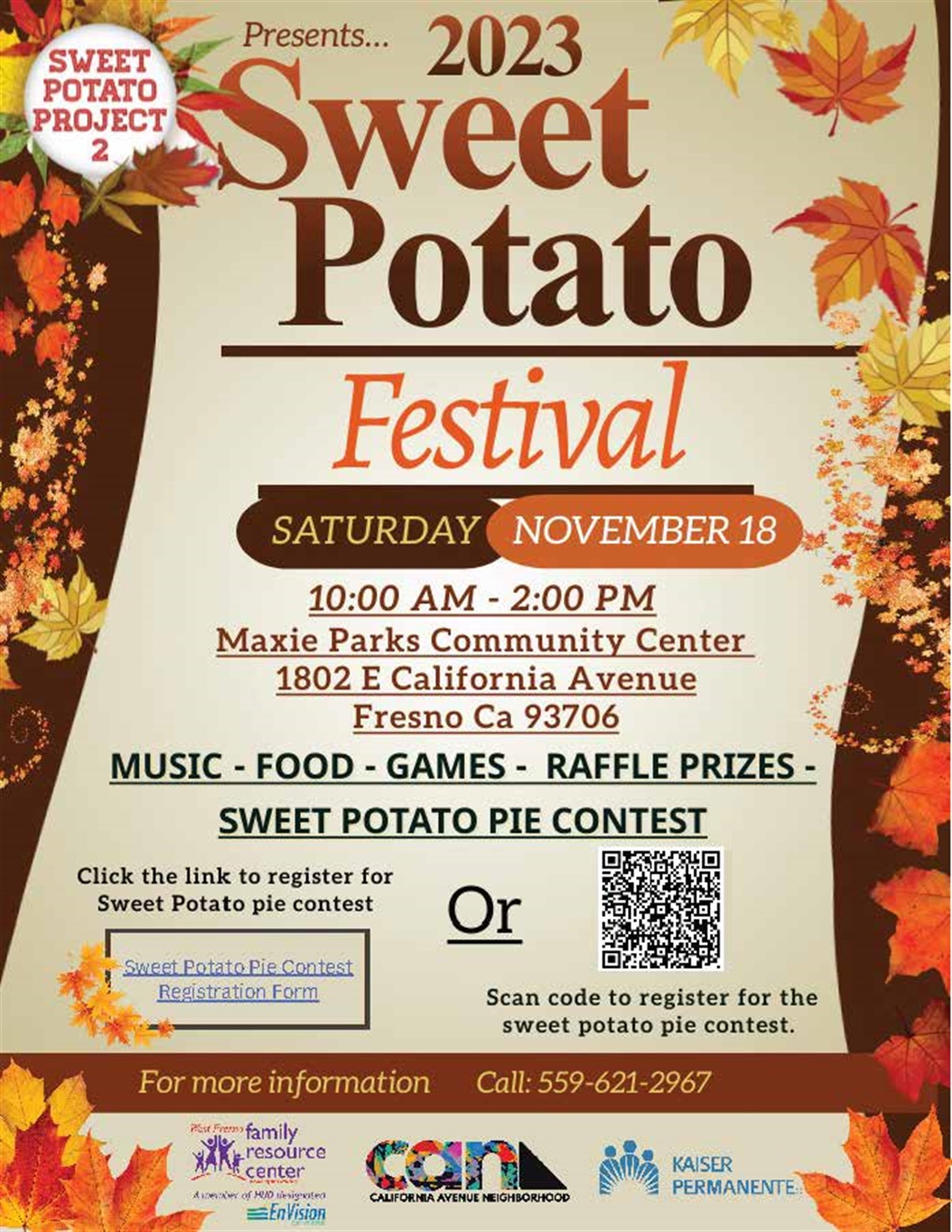The image appears to be a digital flyer for a fall-themed event titled "Sweet Potato Project 2 presents 2023 Sweet Potato Festival." The flyer features a vibrant autumn motif with orange, yellow, and brown leaves adorning the sides, emphasizing a fall aesthetic with a primary color scheme of brown and orange. 

The top of the flyer announces the event details: "Saturday, November 18th from 10 a.m. to 2 p.m. at Maxi Parks Community Center, 1802 East California Avenue, Fresno, California, 93706." The event promises various activities including music, food, games, raffle prizes, and a sweet potato pie contest.

A call to action is present in blue text enclosed within a box, directing attendees to "Click the link to register for the sweet potato pie contest." Alternatively, participants can scan a QR code provided on the flyer for registration. 

At the bottom of the flyer, contact information is provided for further inquiries: "For more information, call 559-621-2967." The logos of the supporting organizations are displayed, including Family Resource Center, CAN California Avenue Neighborhood, Envision, and Kaiser Permanente.

The flyer effectively uses visual elements and provides comprehensive information about the event, ensuring clear communication to potential attendees.